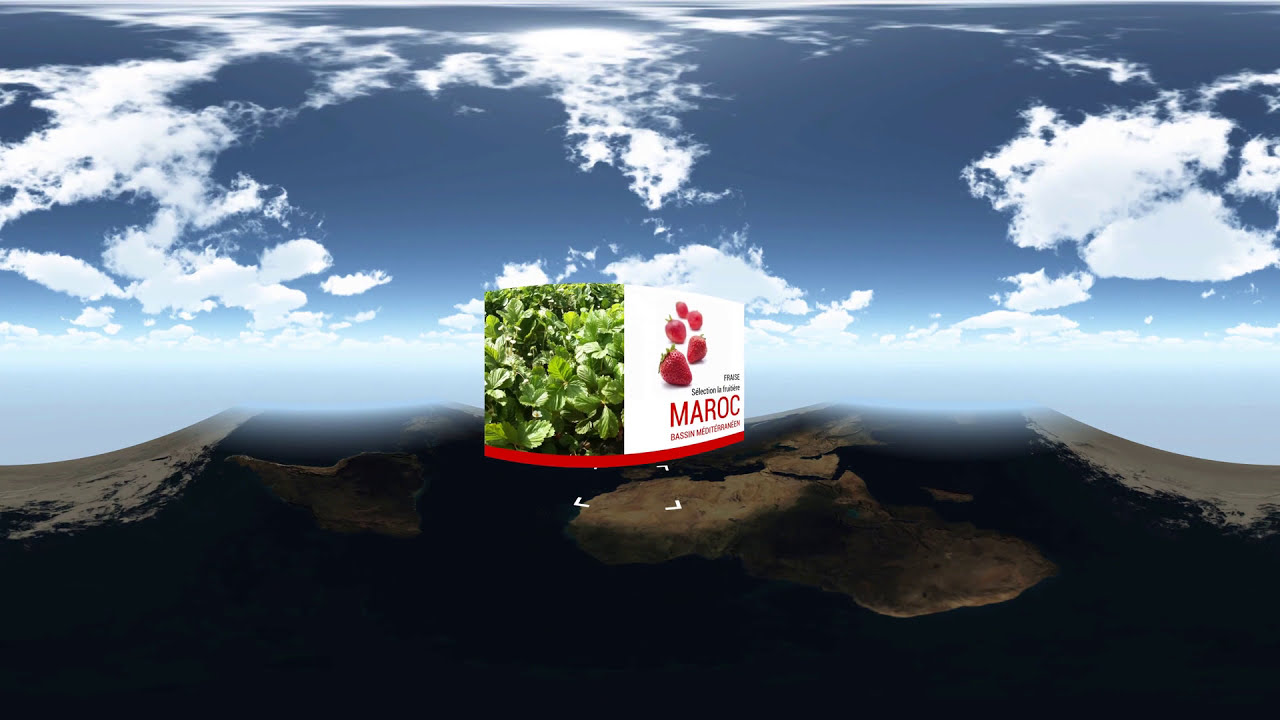The image portrays a surreal landscape blending a photograph and digital rendering. The upper portion showcases a gradient sky, transitioning from dark blue at the top to lighter blue in the middle, streaked with thin, white, wispy clouds. Just below the sky, a layer of fog-like whiteness stretches horizontally across the image. In the lower half, the scene resembles an aerial photograph from space, depicting dark terrains and brown landmasses. A distinct brown landmass occupies the left side, surrounded by dark regions and adjacent white clouds, reminiscent of storm formations seen from space. Another prominent landmass extends from the middle to the right, partially obscured by the central fog-like layer, with more white features to its right, likely signifying clouds.

Dominating the image's center is a digitally rendered cube, slightly tilted to the right, displaying distinct sides. The front side, on the right, features red text spelling "MAROC," above which a cluster of red strawberries is depicted against a white background. The left side of the cube showcases green plants, possibly basil, with a red border along the bottom. Beneath the cube are small white brackets, suggesting the cube has emerged from this frame and might be in motion. This complex, blended artwork appears to be part of an intricate, possibly promotional, digital rendering, yet its exact purpose remains ambiguous.